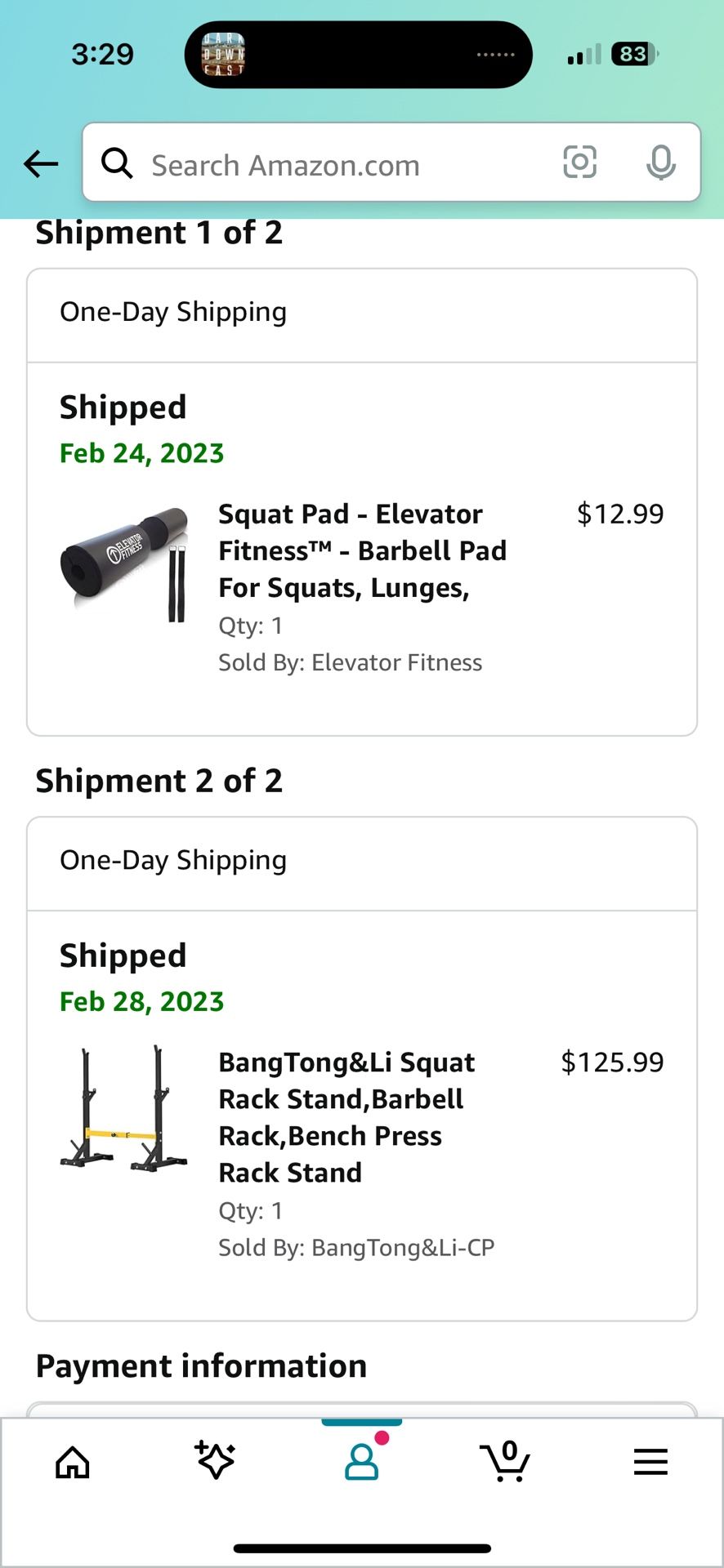The image displays a user's order page on the Amazon mobile application. At the top of the screen, there is a "Search Amazon" box for searching the site. Below this, the order details begin with "Shipment 1 of 2," noting that it has one-day shipping and was shipped on February 24th, 2023. The shipment includes a "Squat Pad from Elevator Fitness," which is a barbell pad designed for squats and lunges. Only one unit was purchased, sold by Elevator Fitness, and the cost was $12.99.

Further down, "Shipment 2 of 2" is detailed, also with one-day shipping and shipped on February 28th, 2023. This shipment contains the "Bangtong and Lee Squat Rack Stand," used as a barbell rack and bench press stand. One unit was purchased, sold by Bangtong and Lee, at a price of $125.99.

Beneath these details, there is a section labeled "Payment Information," but the specific payment details are not visible. At the bottom of the screen, the standard Amazon icons can be seen, including Home, Specials, Profile (which is currently selected), Shopping Cart, and a menu button represented by three horizontal lines for additional options.

The overall interface shows it's 3:29 PM when the user is viewing this page. The user's Amazon profile picture displays a building, and the mobile service indicates two out of four bars of connectivity.